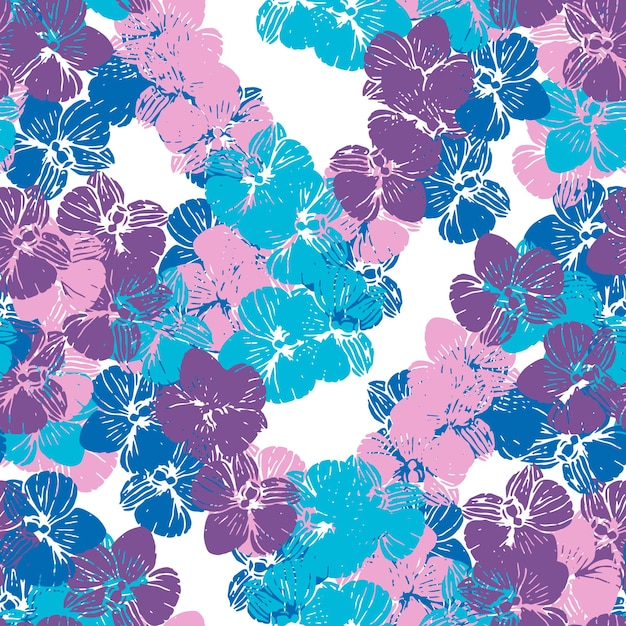This is a digital illustration designed to resemble a repeating pattern, ideal for backgrounds, fabric, or wallpaper. It features stylized hibiscus flowers stamped onto a white background in shades of purple, pink, lighter turquoise blue, and darker navy blue. Each flower has five petals with white inked-out lines and central dots, giving them a clunky, less detailed appearance. The flowers overlap slightly, creating a dense cluster with minimal white space in between. The uniformity and arrangement suggest that the design could seamlessly repeat, enhancing its suitability for various decorative applications.